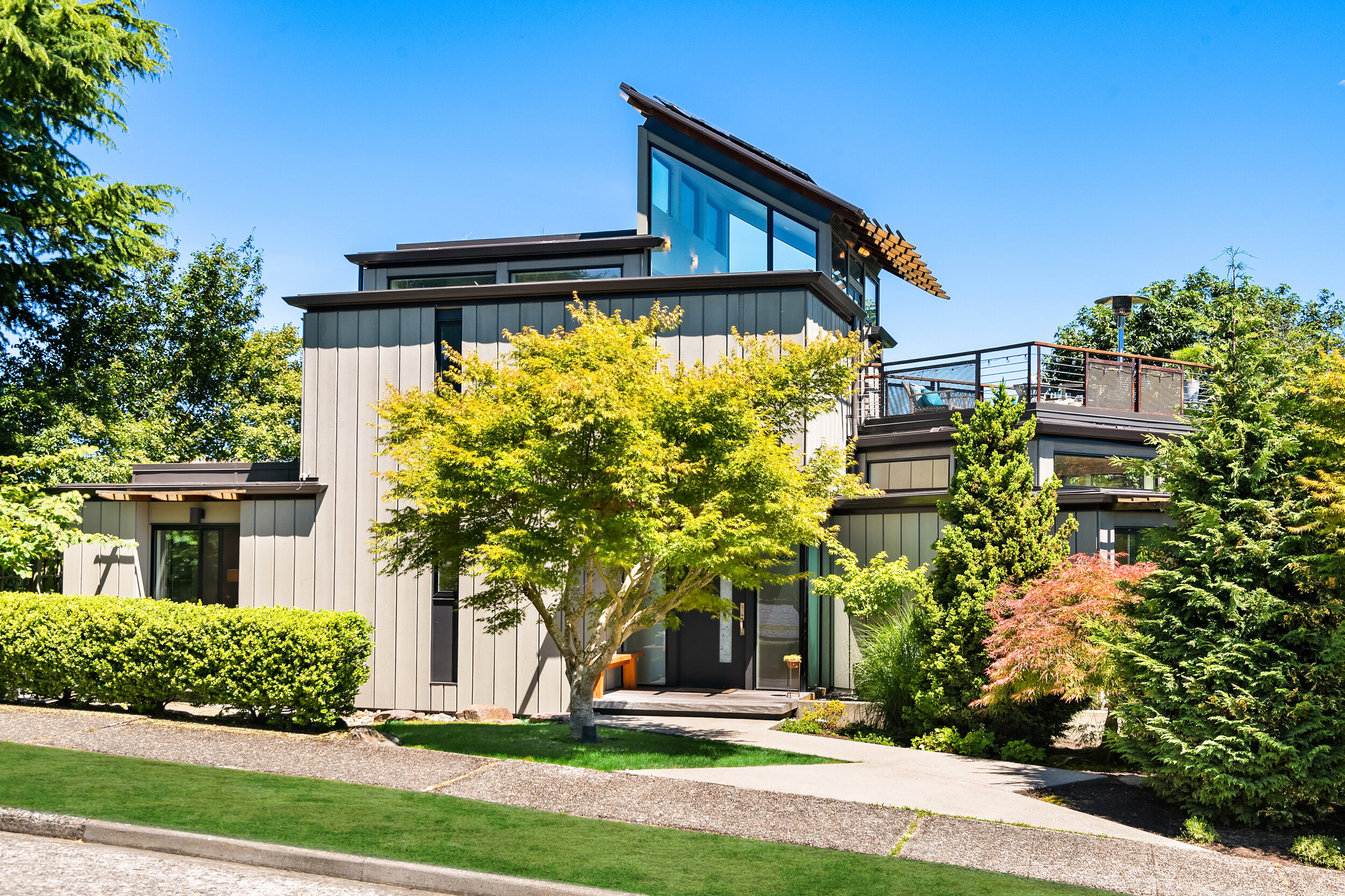This color photograph captures a modern, angular house reminiscent of 70s or 80s architecture, similar in style to the house from the show The Brady Bunch. Taken from the driveway or roadside, the image shows a light gray curb and pavement in the lower left corner, followed by a strip of green grass and a light beige walkway that zigzags into the house. The house has a sand-colored exterior with brown trim and features multiple flat roofs at different levels, a sloped roof with large glass panels, and a rooftop patio on the left side. A tall tree with light green leaves, standing several stories high, dominates the foreground, surrounded by various shrubs, green bushes, and additional trees including evergreens, a little red maple, a pine tree, and more regular trees. An orange bench sits next to the brown front door, and a bright blue sky provides a cheerful backdrop.